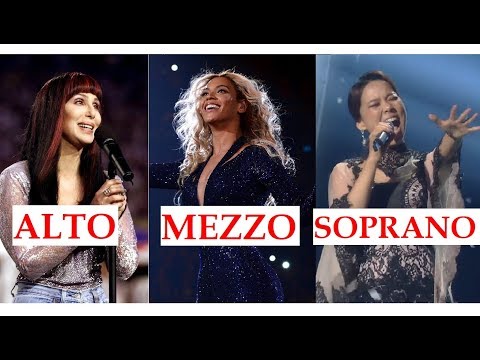The image is a triptych of three photographs, each bordered by a black outer frame and an inner white margin. The photographs feature three female musicians, each framed from the waist up and centered within their respective sections. 

The left photograph, labeled "Alto" in red text within a white rectangle, depicts an older white woman with dark red hair and bangs. She is dressed in blue jeans and a long-sleeve, glittery silver top with a low neckline, holding a microphone stand with a microphone. The woman appears to be singing into the microphone, captured in an expressive moment.

The center photograph, marked "Mezzo" in similar red text, presents a light-skinned Black woman with voluminous blonde hair. She is wearing a black, sparkly one-piece jumpsuit with a deep V-neck. Her joyful smile and upward gaze suggest she is immersed in her performance.

The right photograph, labeled "Soprano," features an Asian woman in an intense performative pose. She wears a sleek black dress and holds a microphone while reaching out with one hand. Her mouth is open, conveying a powerful singing moment.

The photographs, resembling three windows aligned side by side, emphasize the diversity and unique styles of the singers, against the consistent backdrop of the black and white borders.